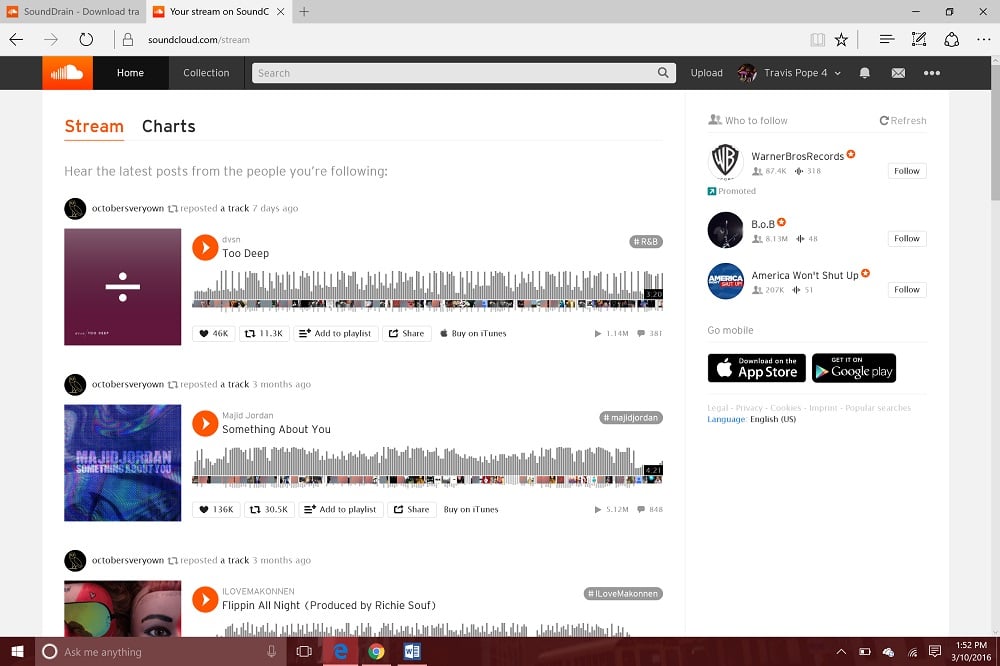This image showcases the desktop version of the SoundCloud browser. The browser interface features a gray top bar with two tabs open on the left: the first titled "Sound Drain - Download" and the second, currently active, labeled "Your Stream on SoundCloud."

The SoundCloud header is a distinctive black bar. On the far left, the recognizable SoundCloud logo is displayed in bright orange. To its right are the main navigation categories: "Home" and "Collection." Centrally located is the search bar, an essential tool for users to explore new tracks. To the right of the search bar, there is an "Upload" button followed by the user's login name. Further right, there are icons for alerts, messages (envelope icon), and a general menu (three horizontal lines icon).

Directly below the header are two primary categories labeled "Stream" and "Charts," with "Stream" currently selected and highlighted in orange. Underneath, the text "Hear the latest posts from the people you're following" appears in small gray font, giving context to the streams below.

The main content area features a vertical list of posts. At the top left of each post is the user's profile photo. Next to this, the user's name is displayed, accompanied by an icon similar to a retweet, indicating that a track was reposted seven days ago.

To the left of the post's middle section is a square thumbnail, which is either an album cover or another graphic. Positioned at the top right of the thumbnail is an orange circle containing a play button. Next to this button, the artist's name and the song title are listed. Stretching across the center is a waveform graph, visually representing the track's audio.

At the bottom of each post listing, there are several interactive icons: hearts for likes, a retweet icon for reposts, an option to add the track to a playlist, a share button, and an option to purchase the track on iTunes. 

This detailed structure allows users to navigate efficiently and stay updated with the latest tracks from their followed artists.